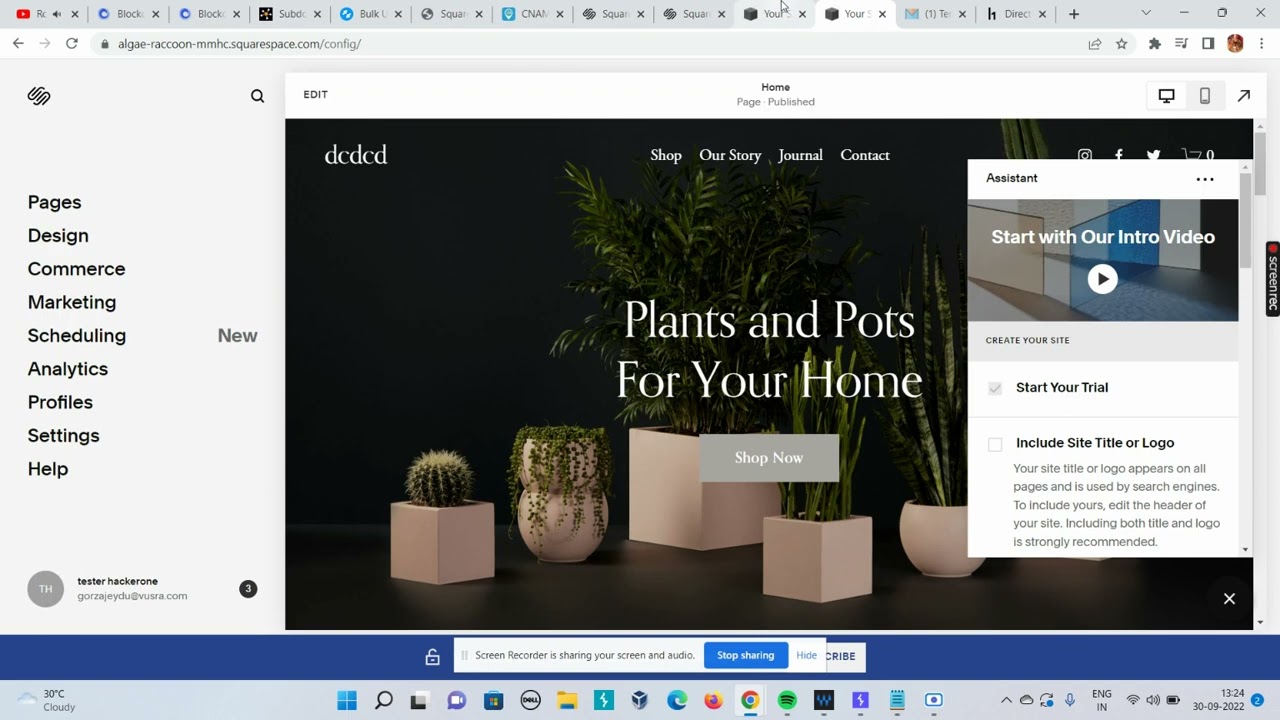A detailed descriptive caption for the image:

---

This image depicts a web browser displaying the configuration page for a Squarespace website, accessible via the URL algae-raccoon-mmhc.squarespace.com/config. The browser window is populated with multiple tabs, including several related to Squarespace alongside other websites.

At the top of the page, the Squarespace interface indicates the webpage being shown is the homepage and is currently published. The central part of the screen features a section with a photograph of potted plants accompanied by the text: "Plant some pots for your home." To the right of this image, a pop-up from the Squarespace assistant provides introductory guidance, featuring options such as "Play Intro Video," "Create Your Site," and "Start Your Trial." The assistant window also includes instructions about adding a site title or logo, emphasizing the importance of editing the site header to include both for better search engine optimization.

At the bottom of the screen, a notification indicates that "Screen Recorder is sharing your screen and audio," with a button labeled "Stop Sharing" to terminate the sharing. The taskbar below this notification showcases several application icons, including a web browser (Chrome), Dell, a file folder, a movie camera icon, a window pane, a magnifying glass, and Spotify, suggesting these applications are currently open.

To the right of these icons, additional system status icons display a microphone, Wi-Fi signal strength, speaker volume, and battery life, implying that the interface is running on a laptop.

To the left of the central plant graphic, the navigation sidebar lists various sections including Pages, Design, Commerce, Marketing, Scheduling, Analytics, Profile Setting, and Help, offering a comprehensive overview of the different configuration options available within the Squarespace platform.